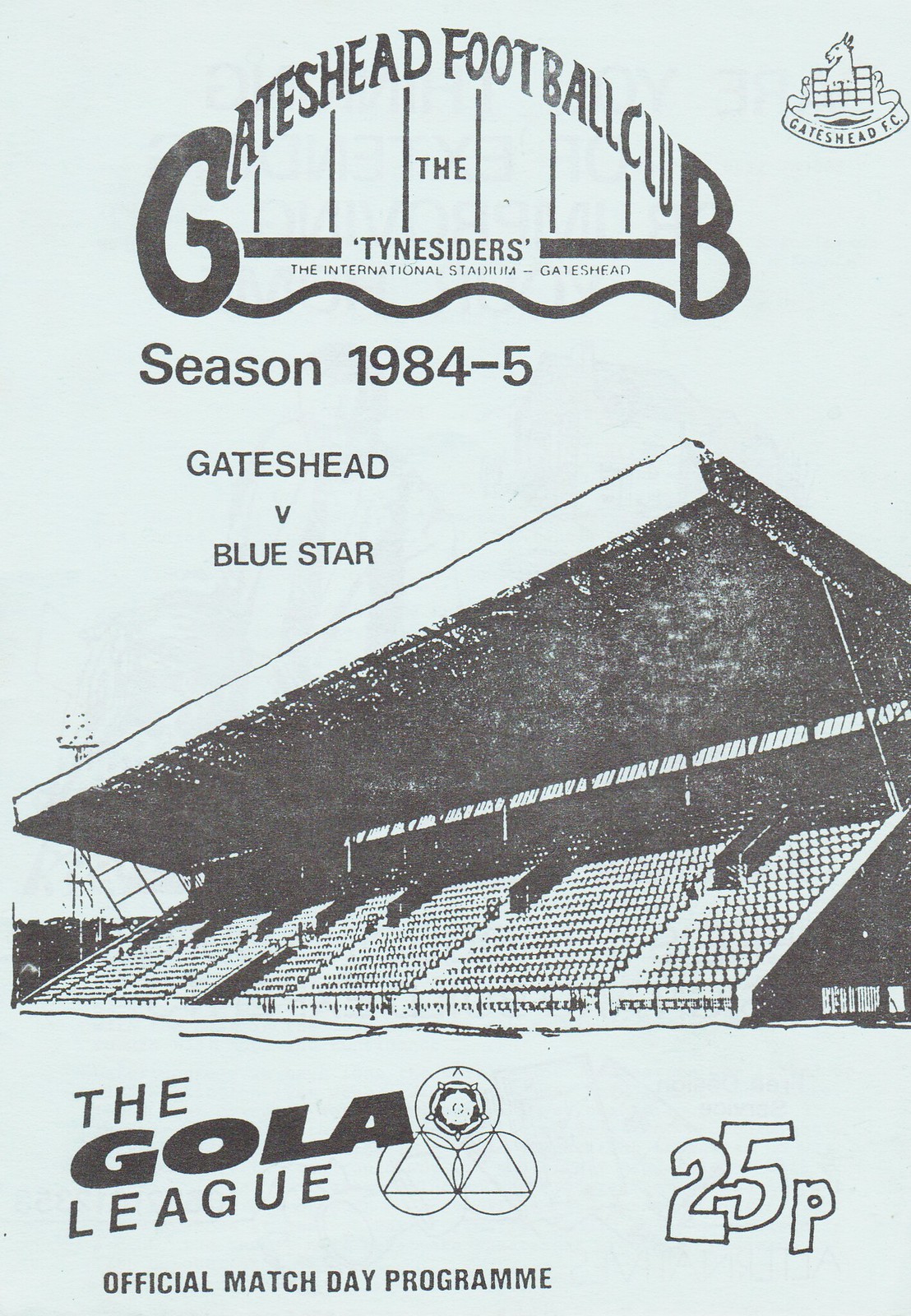The flyer is a vintage piece from the 1984-85 football season, featuring a subdued light blue background with black text and images. At the center is a hand-drawn illustration of an empty grandstand under a roof, with floodlights visible in the distance. The grandstand area has text inscribed on it, adding to the historical feel. Across the top, bold text announces "Gateshead Football Club, the Tynesiders," with "The International Stadium, Gateshead, Season 1984-85, Gateshead vs. Blue Star" directly underneath. In the upper right corner, there is a logo featuring Gateshead Football Club, which includes a distinctive design that appears to be a goat. Near the bottom, standout text reads "the GOLA League" accompanied by a logo with three intersecting circles containing a triangle and a floral or shield-like emblem in the upper angle of the triangle. Below this, the text states "official match day program" with "25p" noted in the bottom right corner.